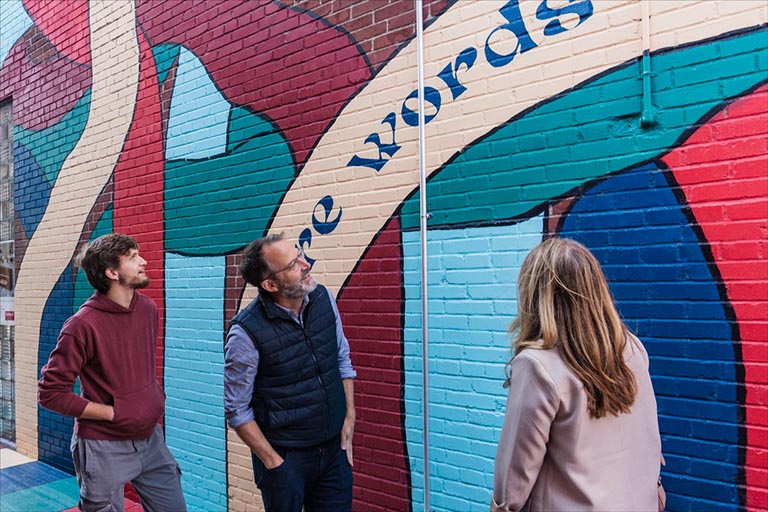The image captures an angled view of three people lined up and gazing at a multi-colored, abstract mural painted on a red brick building. On the left stands a young man with a medium-length hairstyle and a small beard, wearing a burgundy sweatshirt and grey pants. In the middle, an older gentleman in his fifties, with a grey beard, brown hair, and glasses, is dressed in a blue jean shirt with rolled-up sleeves, a blue puffy vest, and dark blue jeans. To the right, a woman with long, blondish-brown hair, facing away and wearing a cream-like grey jacket, completes the scene. The mural they are admiring features a mix of thick, colorful lines in shades of burgundy, teal, baby blue, and red, with a prominent tube-like shape curving from the bottom to the upper right. The mural appears to include the word "words," set against the richly painted backdrop.